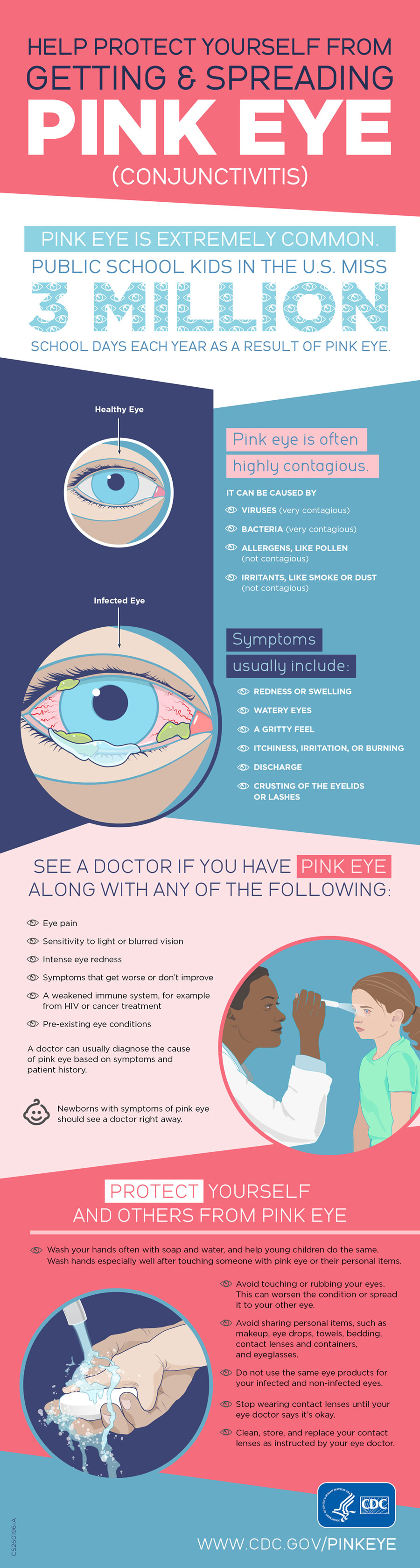This detailed infographic provides comprehensive information on how to protect yourself from getting and spreading pink eye (conjunctivitis). The top section has a dark blue text on a light red background that reads, “Help protect yourself from getting and spreading,” followed by “PINK EYE” in large white bold font, with “conjunctivitis” in parentheses underneath. Below this header, the infographic warns that pink eye is extremely common, noting that public school kids in the US miss 3 million school days each year due to the condition. 

The infographic is segmented into various polygonal shapes, with sections featuring images and information. To the left is a comparison image showing what a healthy versus an infected eye looks like. Next to it, it elaborates on the contagiousness of pink eye, mentioning that it can be caused by viruses and bacteria (both very contagious), allergens like pollen (not contagious), and irritants like smoke or dust (not contagious). Symptoms are outlined in detail and include redness or swelling, watery eyes, a gritty feeling, itchiness, irritation or burning, discharge, and crusting of the eyelids or lashes.

Below the symptom section, there is advice on when to see a doctor if you have pink eye, illustrated with an image of a doctor examining a little girl's eye. The bottom part of the infographic offers suggestions on how to protect yourself and others from pink eye, highlighted by an image of someone washing their hands. The website www.cdc.gov/pinkeye is cited at the very bottom for further information.